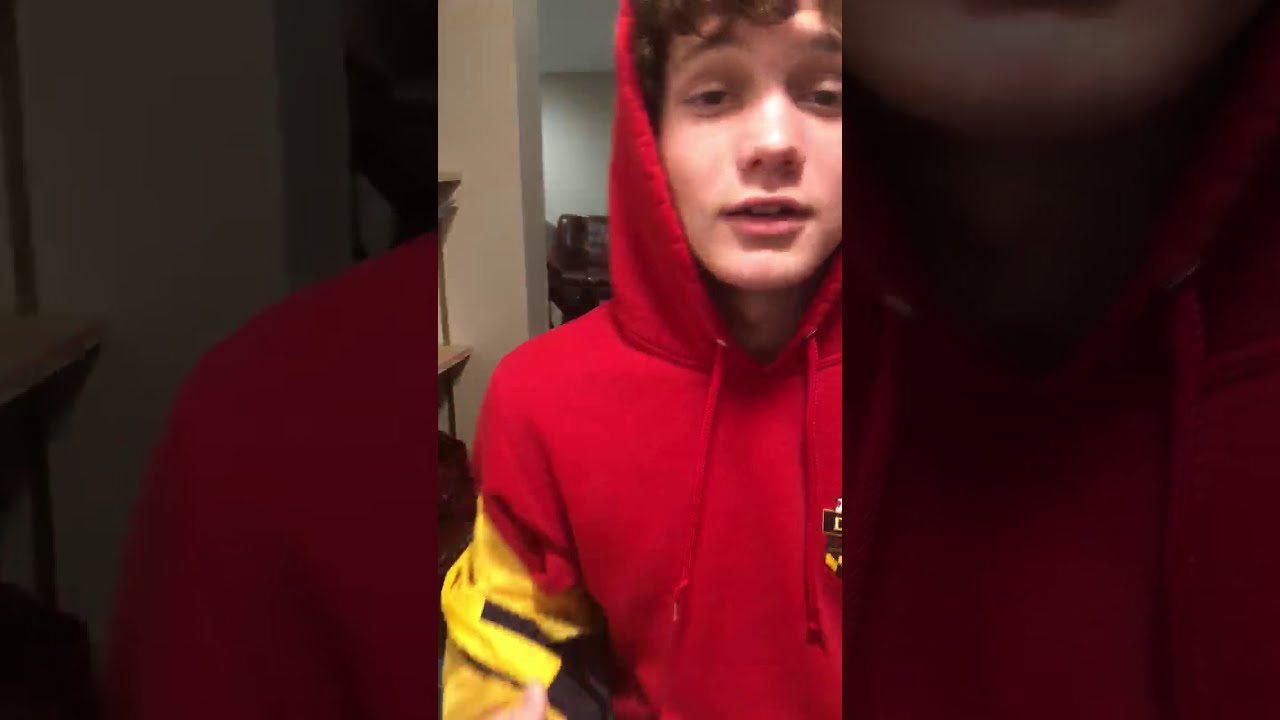A teenage boy, approximately 14-15 years old, is the main subject of this image. He is standing slightly off to the right side, taking a selfie while looking directly at the camera. He is dressed in a red hoodie with the hood up, featuring yellow sleeves and red drawstrings dangling below his chin. There is a partially visible crest on the left side of his chest. The boy has dark, curly hair peeking through the front of the hood, and his dark eyebrows and slightly squinted eyes give him a focused expression. He has a typical straight nose, and his mouth is slightly open, revealing his top teeth. The background suggests an indoor setting, possibly a room in a house, with visible elements like a white wall, a couple of shelves, and a doorway through which a brown chair and a table can be seen. The colors in the image include various shades of yellow, red, brown, tan, and pink. The style of the photo hints that it could be a screenshot from a mobile app like TikTok or Instagram, with some areas of the image slightly magnified and tinted, particularly around the edges.